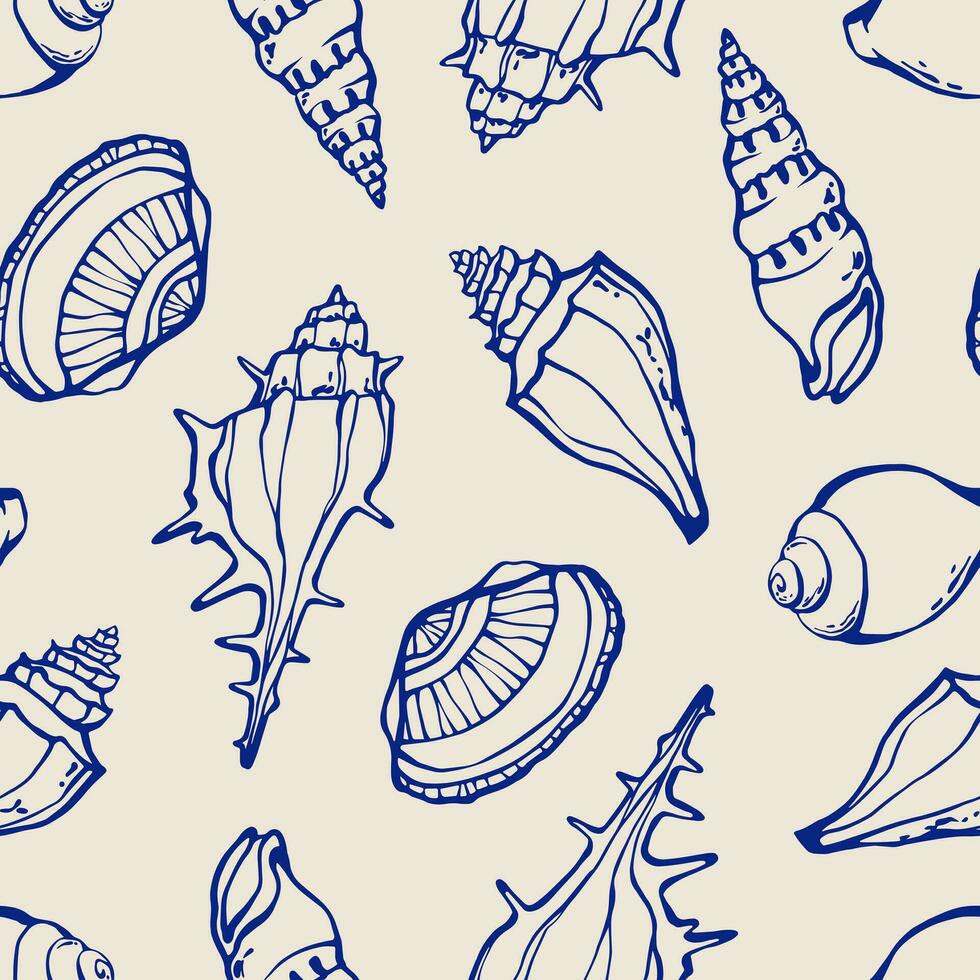This image features a wallpaper sample with a subtle off-white or whitish-gray background adorned with a captivating assortment of seashell illustrations in navy blue ink. The shells, meticulously outlined with some accentuated features, are scattered across the wallpaper in various orientations, contributing to a random but harmonious pattern. The assortment includes a diverse range of seashells typically found at the beach, such as large conch shells, scallop shells, and smaller, intricately spiraled snail shells. There's notable space between each shell, ensuring they don't overlap, and their sizes vary, with larger conch shells and smaller spiky or fan-like shells adding to the visual interest. The simplicity and elegance of the design make it versatile for use as wallpaper for a room or even as a phone background, capable of spreading seamlessly across larger surfaces when multiple squares are connected.